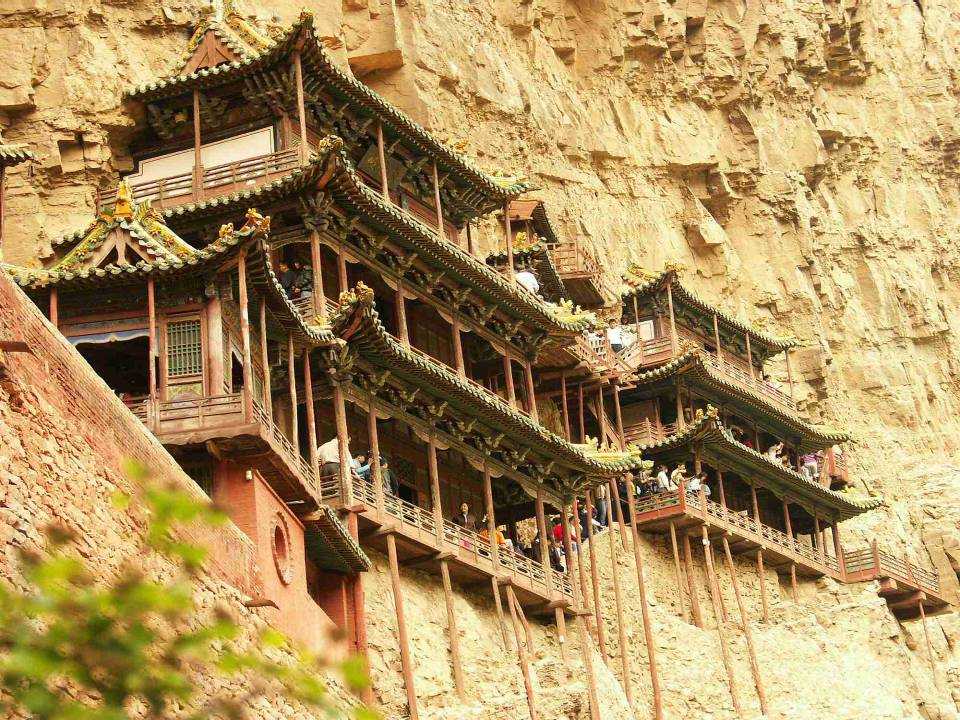This image features a stunning depiction of traditional Japanese-style architecture uniquely built into the side of a rugged, clay-colored mountain. The structures appear to be three stories high, displaying a beautiful blend of ornamental and practical design elements that speak to an old-world quality. The buildings, protruding slightly from the vertical rock wall, are adorned with intricate, rounded roof tiling in green and yellow tones, and angular awnings with triangular tops.

Supporting wooden poles run into the rock wall, reinforcing decks and long porches where many people can be seen standing, sitting, and gazing out into the distance. The facades of these buildings show a combination of clay-colored stone and brick, merging seamlessly with the natural environment. Detailed ornate trimming embellishes the roofs, adding to the structure's elaborate aesthetic.

The mountain itself is marked by numerous crevices and patches of greenery sprouting from its sides, with some clusters of green and yellow bushes visible in the bottom left corner of the image. This blend of majestic natural landscape and refined architecture captures the essence of a foreign land, likely Japan or China, where ancient design meets the dramatic natural elements of a cliffside.